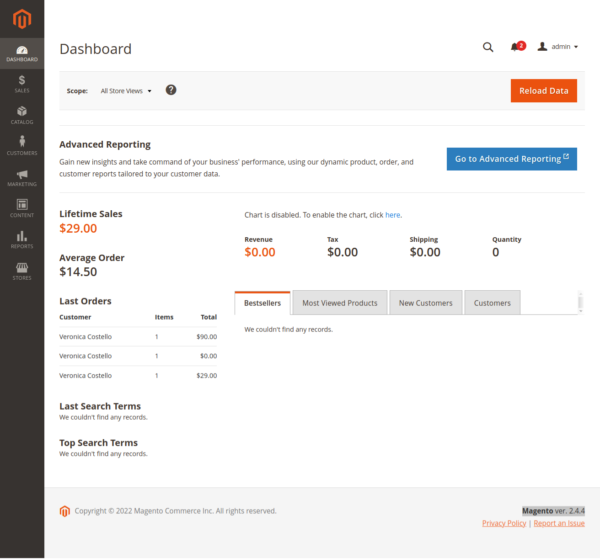The image showcases a detailed view of a website's admin dashboard. The interface features a black sidebar on the left side of the screen that runs vertically from the top to the bottom. At the top of this sidebar is a red graphic, beneath which a vertical menu is displayed. The menu options listed are: Dashboard, Sales, Catalog, Customers, Marketing, Content, Reports, and Stores.

The background of the main section of the dashboard is an off-white, stone-like texture. At the top center of the screen, the word "Dashboard" is prominently displayed in capital letters. Moving to the right, there are icons for a magnifying glass, a notification bell with a red circle indicating two new notifications, and a silhouette of a person representing user profile access. Next to this icon is "Admin" in lowercase letters, accompanied by a drop-down arrow.

Below this, a light gray banner stretches across the width of the dashboard. This banner contains a drop-down labeled "Scope: All Store Views" and a circle with a question mark symbol inside it for help or additional information. On the far right of this banner, there is a "Reload Data" button with white text.

The content below the banner introduces "Advanced Reporting" with the tagline, "Gain New Insights and Take Command of Your Business' Performance Using Our Dynamic Product, Order, and Customer Reports Tailored to Your Customer Data." A blue button labeled "Go to Advanced Reporting" with white text invites users to access the advanced features.

Further down, the dashboard displays "Lifetime Sales" in orange text with a value of $29, and "Average Order" in black text with an average value of $14.50. Additional sections include headers for "Last Orders," "Last Search Terms," and "Top Search Terms."

A notice states, "Chart Is Disabled. To enable the chart, click here," with the word "here" in blue text as a hyperlink. Financial metrics such as "Revenue $0," "Tax $0," and "Shipping $0" are also listed, along with "Quantity $0."

The "Best Sellers" section is highlighted with a white background and an orange line at the top. Adjacent sections include "Misused Products," "New Customers," and a general "Customers" section, both identified by their gray headers.